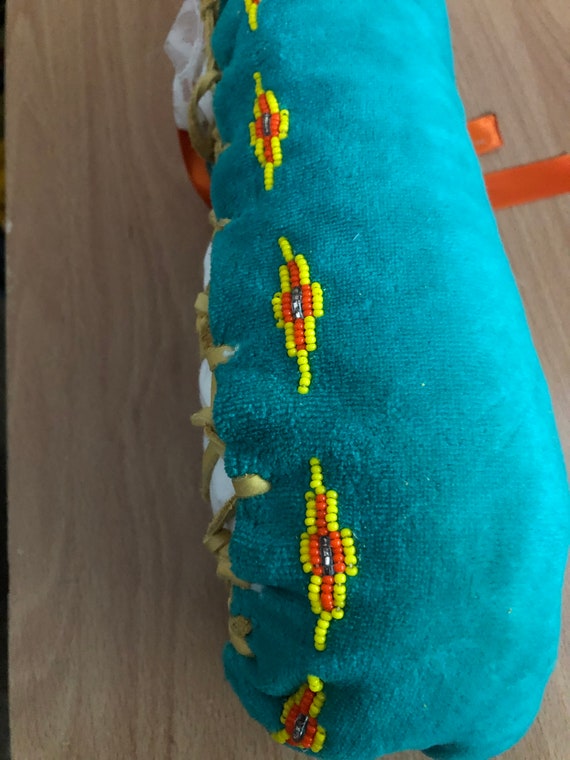The photograph showcases a close-up view of a brightly colored, tubular-shaped fabric object, possibly part of a stuffed animal or a sewn garment like a sweater sleeve, laid out on a light-colored, faux woodgrain table. The fabric is a vibrant turquoise, which appears soft and fuzzy, reminiscent of a sweater or blanket material. The focal point of the object features elaborate hand-beading in an intricate Native American style. The beadwork forms a striking diamond pattern: at the center are gray or silver beads surrounded by orange beads, which are encircled by bright yellow beads, all tiny and meticulously sewn onto the turquoise fabric. Additionally, there's visible gold ribbon stitching on the left side. An orange ribbon lies on the table behind the object, and some white fabric with brown lacing peeks out from underneath, adding to the intricate detailing.